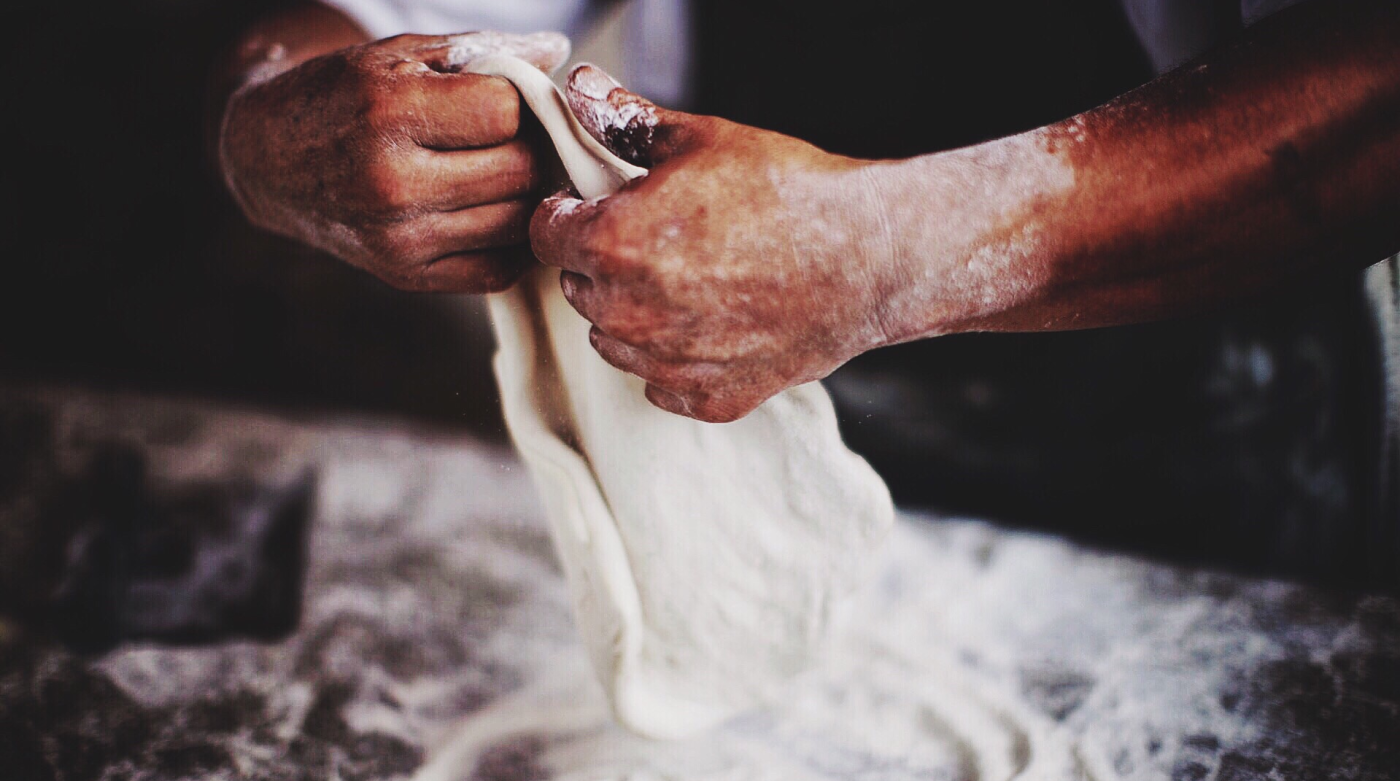The photograph captures a close-up, artistic view of a pair of well-worn, aged hands, deeply tanned and dusted with flour, skillfully shaping a circular piece of pizza dough. The hands, fingers curled and grasping the dough tightly, work together to stretch and flatten it further, holding it aloft over a dark, likely marble countertop generously covered with scattered flour. The composition of the image suggests an intimate and focused moment, with the background blurred, providing a stark contrast that highlights the textures and details of the weathered hands and airy dough. In the faint background, there is a hint of white, possibly an apron, suggesting a kitchen setting dedicated to the art of pizza making. The photograph's rectangular frame emphasizes the horizontal spread of the scene, drawing attention to the dexterity and experience embodied in the hands.